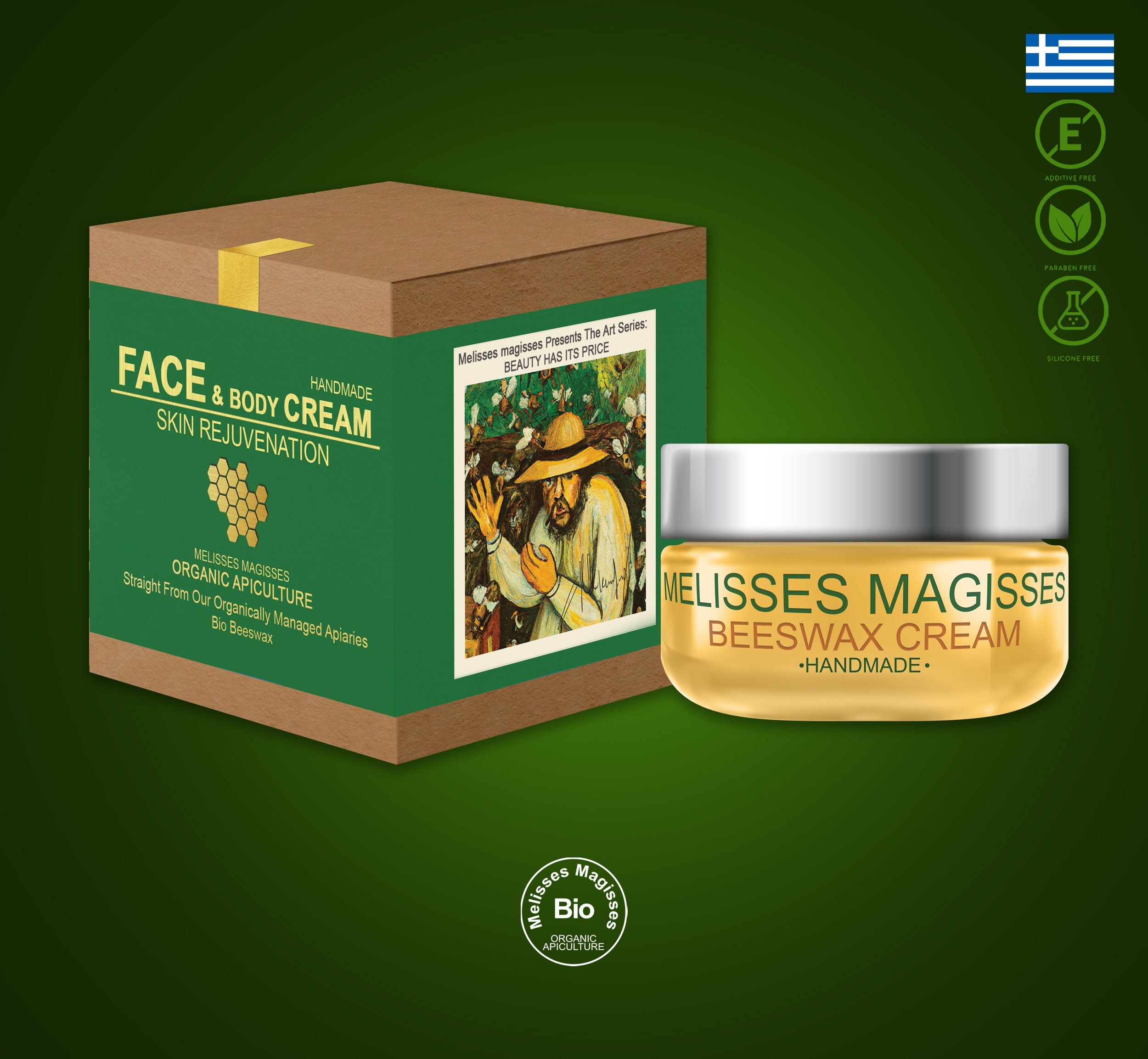In this image, the focus is on a product presented by Melissa's Majesty's Bio-Organic Apiculture. On the left side of the image is a green background with a cardboard box displaying the product. The box features a honeycomb logo in shades of brown and tan, indicating its organic nature. It states "Face and Body Cream" and "Handmade Skin Rejuvenation," highlighting that the cream is crafted with bio-beeswax sourced from organically managed apiaries. The box also includes various certification symbols such as additive-free (E crossed out), paraben-free (leaf icons), and silicone-free (chemical vial crossed out). 

The right-hand side of the image shows a silver-lidded, yellow beeswax cream container. There’s an illustration of a person wearing a sun hat surrounded by bees with a caption that reads, "Beauty has its price,” emphasizing the natural and artisanal quality of the product. Additionally, a Greek flag in the top right corner indicates the origin. This detailed backdrop and packaging suggest the product's commitment to eco-friendly, natural skincare without harmful chemicals.